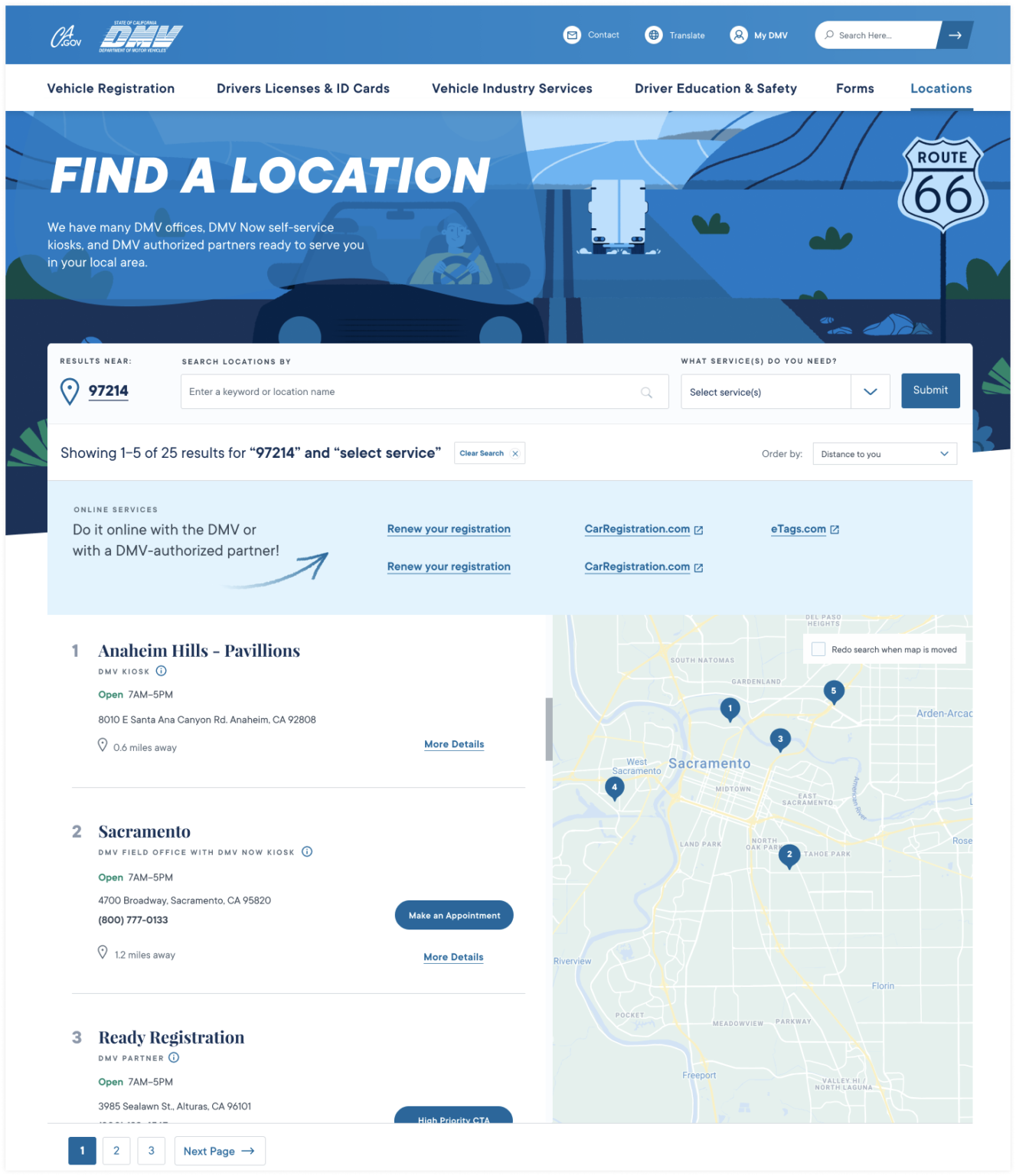The image vividly displays a white banner stretching across the screen, prominently featuring several navigational options: "Vehicle Registration," "Driver's Licenses and ID Cards," "Vehicle Industry Services," "Driver Education and Safety," "Forms," and "Locations." The "Locations" option is currently selected.

Dominating the screen is a large visual of a person driving a car along a road marked as Route 66, situated on the right-hand side. On the left, there's bold white lettering that reads, "Find a Location." Below this header is a search bar where users can input keywords or locations to tailor their search for specific services related to their car. Accompanying the search bar is a submit button for initiating the query.

Beneath this section, five out of a total of 25 search results are displayed, listed sequentially on the left side of the screen. Adjacent to each listing, there is a "Make an Appointment" button, enabling users to schedule appointments with their chosen locations. To the right of the search results, an integrated map visually pinpoints where these locations are situated, providing a comprehensive and user-friendly interface for finding and booking vehicle-related services.